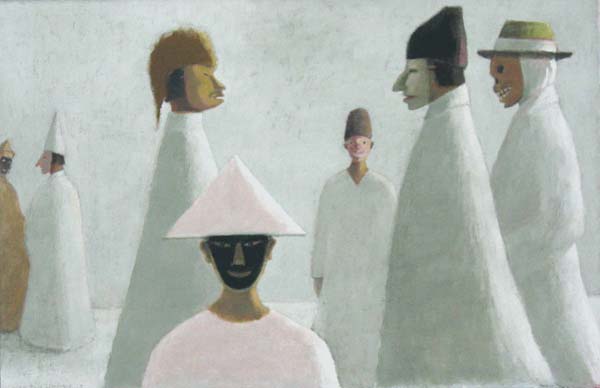The image is an abstract painting featuring seven human figures, all dressed in long white robes that extend to the ground, with their arms barely visible through the sleeves. Each figure wears a unique and varied mask, along with different types of hats, adding to their mysterious and somewhat eerie appearance. The background and floor of the painting are pure white, contributing to the overall monotone color scheme, which is punctuated by shades of beige, light green, tan, brown, pink, gray, black, and white.

Positioned throughout the image, we see:
- To the far right, a man with a skeleton mask and a yellow-and-white fedora hat.
- Directly in front of him stands another man, wearing an Egyptian pharaoh hat and a different styled mask.
- On the back left, a figure in a golden robe with a black mask and gold pointed hat is noticeable.
- Moving to the center, a man donned in a white robe has a golden mask and hat.
- In the foreground towards the center-left is a man with a pink bust and a triangle-pointed hat along with a black mask.
- On the left side, another character wears a white-pointed hat and a pink face mask with a long nose.
- Lastly, two men in the background on the left side add to the composition with their distinct headdresses and masks.

The masks themselves vary in shapes and expressions, some appear to be smiling while others look scary, enhancing the surreal and abstract nature of the painting. The entire image exudes a sense of uniformity through the white robes, yet a striking individuality through the distinct masks and hats.